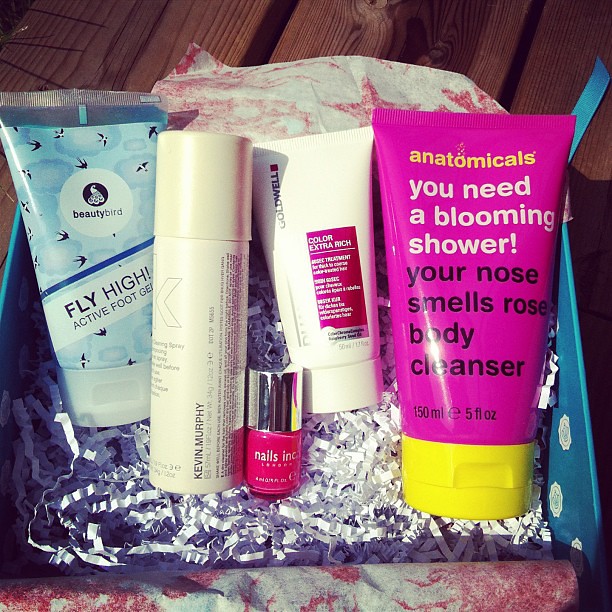The image shows an aqua blue cardboard box with white snowflake-like patterns, positioned on a wooden surface. Inside the box, nestled among white crinkled paper shavings, are several beauty products neatly arranged for display. The first product on the left is a light blue squeeze bottle adorned with black bird motifs and a white circle label featuring a small bird illustration; it is identified as Beauty Bird's "Fly High Active Foot Gel." Next to it, a slender, elongated white bottle from Kevin Murphy is turned sideways, making the exact product name unreadable. Adjacent to this is a bottle of nail polish from Nails Inc., in a vibrant red shade with a shiny chrome cap. Positioned beside the nail polish is a white tube labeled "Color Extra Rich Treatment" from Goldwell, with a pink rectangular highlight on the tube. The final item in the box is a large pink-purple squeeze bottle with a greenish-yellow cap, from Anatomicals, bearing the playful label "You Need a Blooming Shower, Your Nose Smells Rose Body Cleanser."